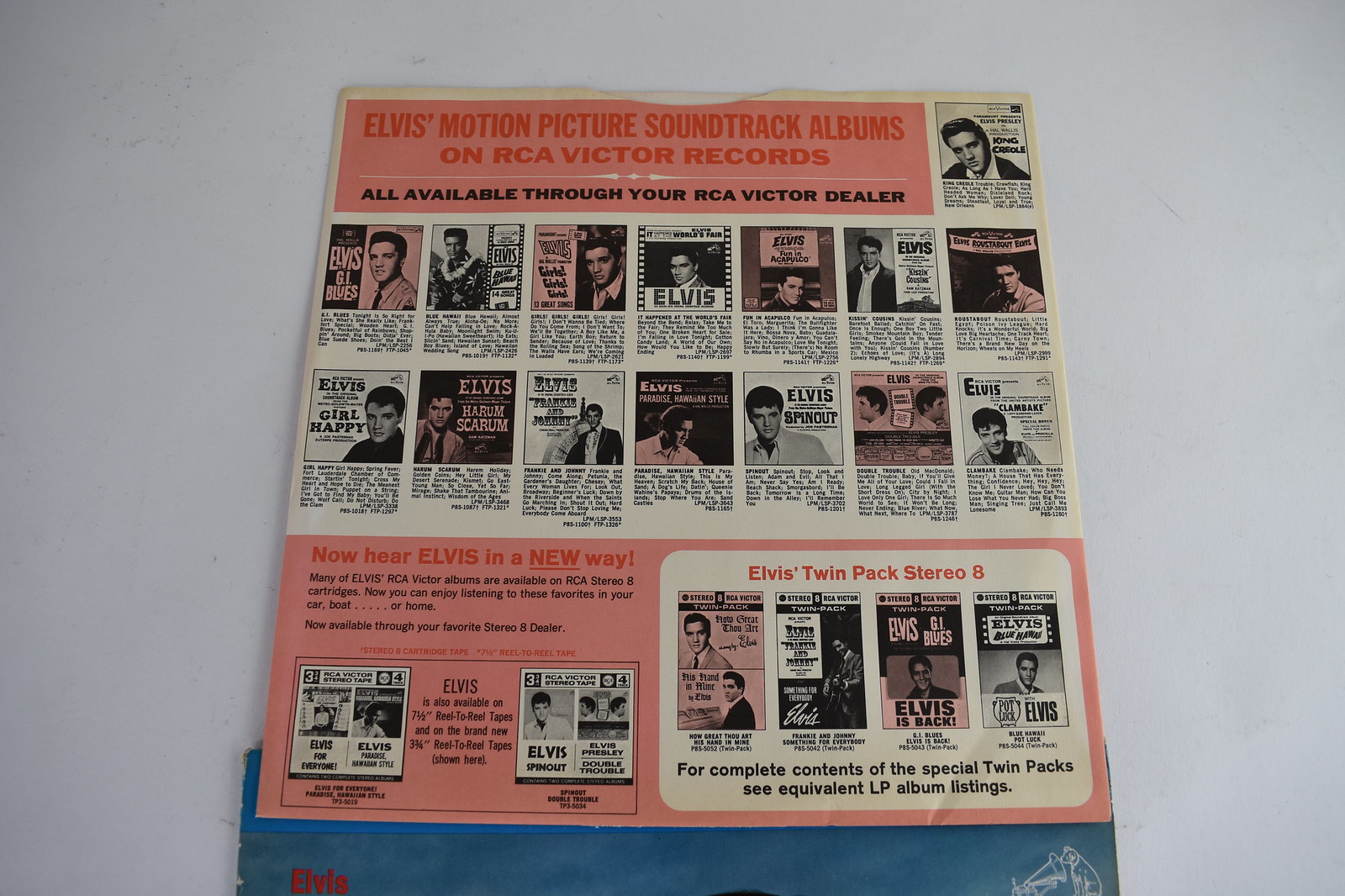The image is an advertisement for Elvis Motion Picture Soundtrack Albums on RCA Victor Records, set against a light gray background. Predominantly salmon pink in color, the ad features a bold pink rectangle at the top with red lettering proclaiming, "Elvis Motion Picture Soundtrack Albums on RCA Victor Records." This banner is followed by a listing of several Elvis albums, totaling around 15. The thumbnailed images of the album covers are arranged in two rows on a lighter background, while below them there are additional thumbnails displayed in a white rectangle located in the bottom right quadrant and a box in the lower left corner. The album covers are depicted in shades of pink, white, and gray, rather than their original colors. The ad also includes another banner at the bottom that reads, "Now Hear Elvis in a New Way," highlighting the Elvis' Twin Pack Stereo 8, along with a few other albums. This advertisement likely originates from a record store setting that sells RCA Victor records.